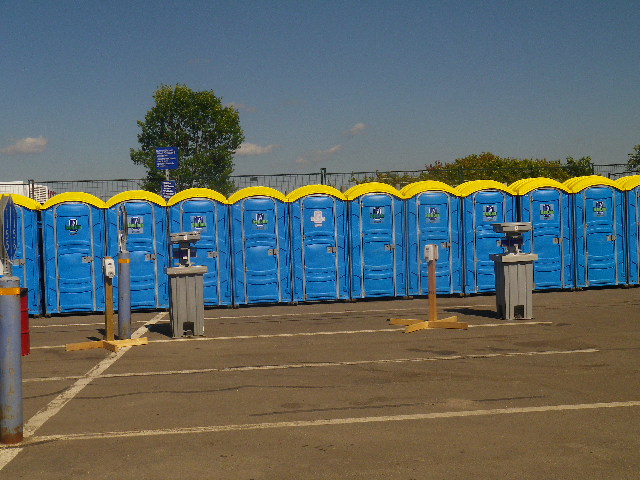In the image, there is a neat row of over 10 bright blue porta potties with distinctive banana yellow roofs, lined up side by side in a large parking lot. In front of the porta potties, there are two freestanding, gray handwashing stations that resemble trash cans, and next to these are wooden stands mounted with small, white sanitizer dispensers. The parking lot is marked with white lines indicating several parking spots, four of which are visible and the fifth obscured by the porta potties. In the middle of the row, one porta potty is different with a white sign rather than the usual green or blue ones, and has stainless steel struts arcing around its front. In the background, there is a tall black fence with vertical poles, beyond which several green trees are visible. The sky above is mostly clear with a few light clouds. Additionally, there is a blue sign with white writing and a stainless steel pole located towards the left side behind the porta potties.